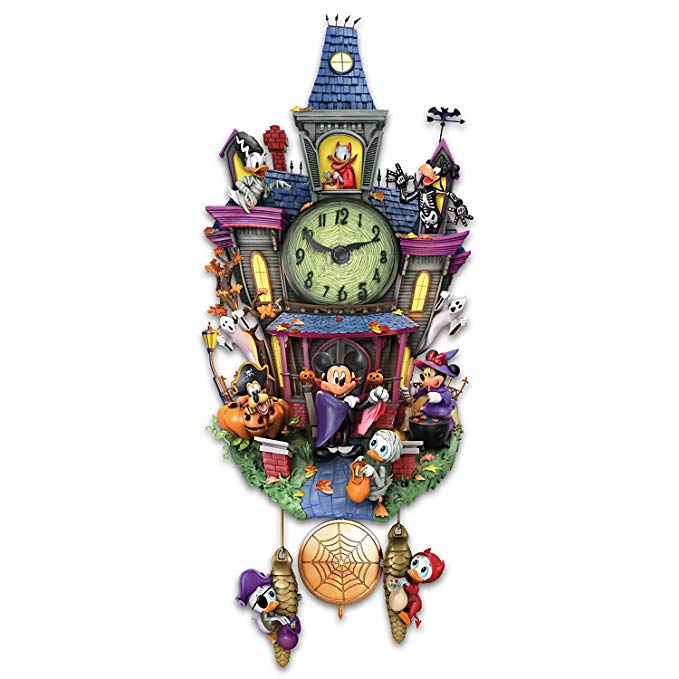This digital rendering features an intricate Disney-themed wall clock, styled like an old-fashioned cuckoo clock with a festive Halloween twist. The clock tower structure showcases various beloved Disney characters in whimsical costumes, adding to the spooky yet playful ambiance. Central to the image is the clock face, around which the characters are arranged.

At the pinnacle of the clock, there's a window where Donald Duck appears sporting devil horns. To the right of the clock face, Goofy can be seen dressed in a skeleton costume. On the left side, a character resembling Marge Simpson's hairstyle can be spotted, although likely intended to be Daisy Duck dressed as the Bride of Frankenstein. Mickey Mouse, dressed as a vampire, stands prominently at the doorway below the clock face, adding to the eerie charm.

Beneath the clock, two weights dangle, each with one of Donald's nephews—Huey and Dewey—hanging from them. The clock also features additional Disney characters decked out in Halloween costumes, pumpkins, and trick-or-treaters, enhancing its festive decor. A web design adorns the bottom section, completing the spooky funhouse effect. This delightful clock captures the essence of Halloween through its enchanting Disney character portrayals and intricate, festive design elements.